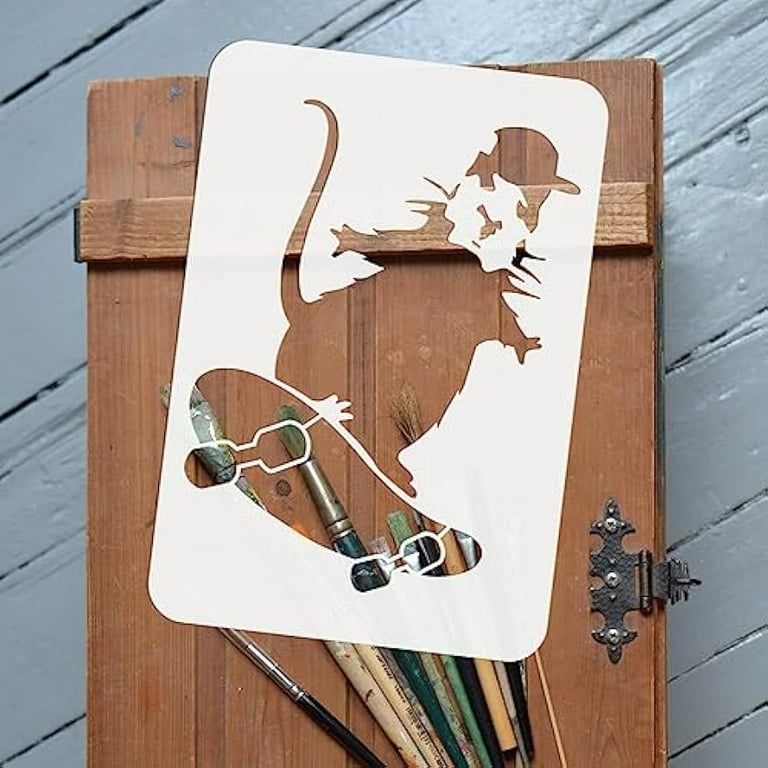The image depicts an artistic setup where a white stencil, featuring a caricature of a rat or hamster wearing a baseball cap and riding a skateboard, is prominently laid on a brown wooden panel. This panel rests on a background of grayish, weathered wooden slats that resemble an old wood shutter, complete with an iron hinge visible about three-quarters of the way down. Adding depth to the scene, a collection of various colored paintbrushes are scattered underneath the stencil, with their bristles pointed at an angle. The overall setting gives the impression of a workspace where someone is preparing to create stencil art on the wooden panel.